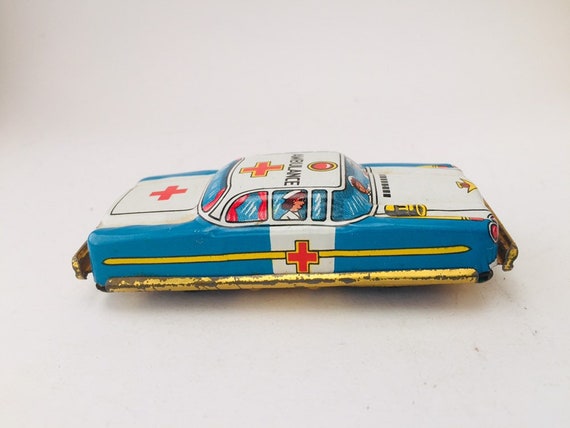The image showcases a close-up of a vintage toy ambulance displayed against an off-white background. The toy itself exudes a worn and aged charm with noticeable rust and chipped paint, indicative of its extensive use over the years. Crafted in the style of the 1950s, possibly originating from post-war Japan, the ambulance features a distinctive, rectangular design with a slightly elevated cabin area.

The sides of the toy are painted blue with a horizontal yellow stripe running across the center. Vertical white square lines accentuate the blue sides, while golden trim embellishes the front, rear bumper, and side panels. A red cross emblem is prominently displayed in multiple locations: on the hood, the top of the cabin, the rear of the car, and within the white area of the sides. The top of the vehicle is white with scattered yellow spots and a yellow logo at the front. "AMBULANCE" is inscribed in black letters across the top.

Inside the model, a Caucasian nurse figure with dark hair, dressed in a white shirt and hat, can be seen positioned centrally behind the windows. Another nurse is visible through the front windshield. The rear window is adorned with red curtains, adding to the ambulance's authentic details. A yellow siren is situated at the vehicle's front. The intricate design and nostalgic wear make this toy ambulance a poignant relic of its era.